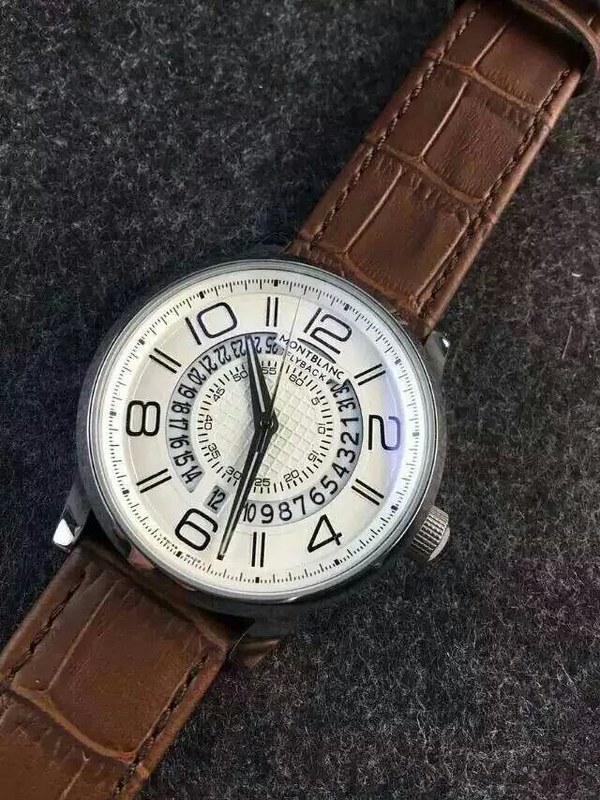This is a close-up photograph of a sophisticated Montblanc Layback wristwatch, carefully placed on a dark gray fabric surface. The wristwatch sports brown leather straps with square paneling, extending diagonally to the top right and bottom left corners of the image. The face of the watch is white, encased in a black frame. The watch displays multiple layers of black numbers: larger ones around the edge, and progressively smaller ones in concentric circles towards the center, giving it a unique and intricate appearance. The black hands, including a black second hand, are set to around 10:25. You can also spot the silver dial on the side used for winding and setting the time. The brand name "Montblanc" and the word "Layback" are prominently visible near the 12 o'clock mark on the clock face.